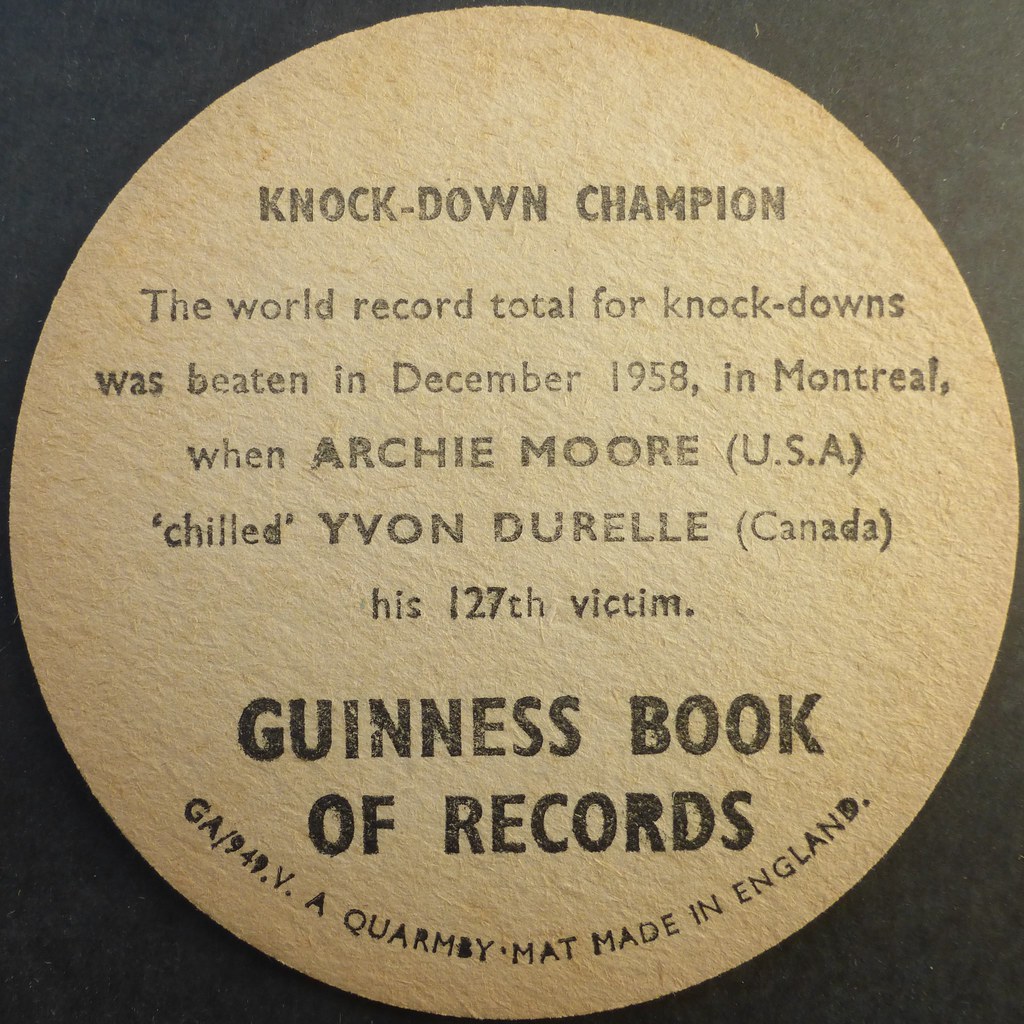The image depicts a circular plaque, resembling a coaster or a sign, with the inscription "Knockdown Champion" at the top. The text details a world record achievement, stating: "The world record total for knockdowns was beaten in December 1958 in Montreal, Canada, when Archie Moore from the USA defeated Yvon Durelle, Canada, marking his 127th victim." Below this, in bold black letters, it reads "Guinness Book of Records." The plaque is brown with black text and bears additional technical information: "GA/949.V.A Quarambi, MAT, made in England." The background of the image is black, enhancing the visibility of the yellow and black-lettered plaque.